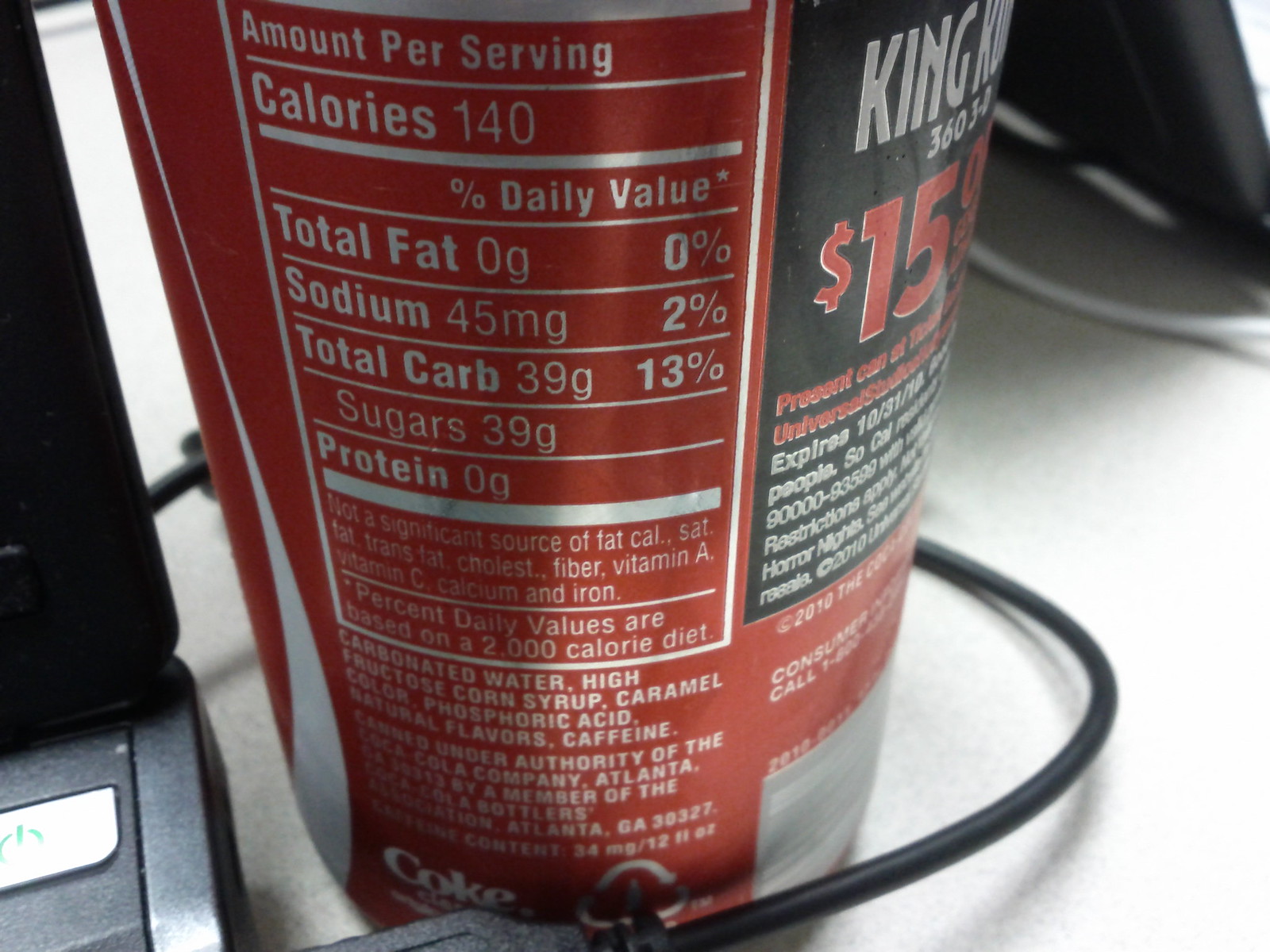The photograph captures a close-up view of a Coca-Cola can prominently displaying the nutrition facts and ingredients label. The can is placed on a gray desk surface. To the left of the can, there's a partial view of an open laptop with its power button visible, and a cord that loops around the can. The can itself is a distinctive red with the iconic Coca-Cola logo in white lettering in the bottom left corner. Additional text on the can is in a silver-white font. On the right side of the image, a black advertisement and a white barcode can be seen. In the top right corner, part of a desk phone is visible, completing the workspace setting.